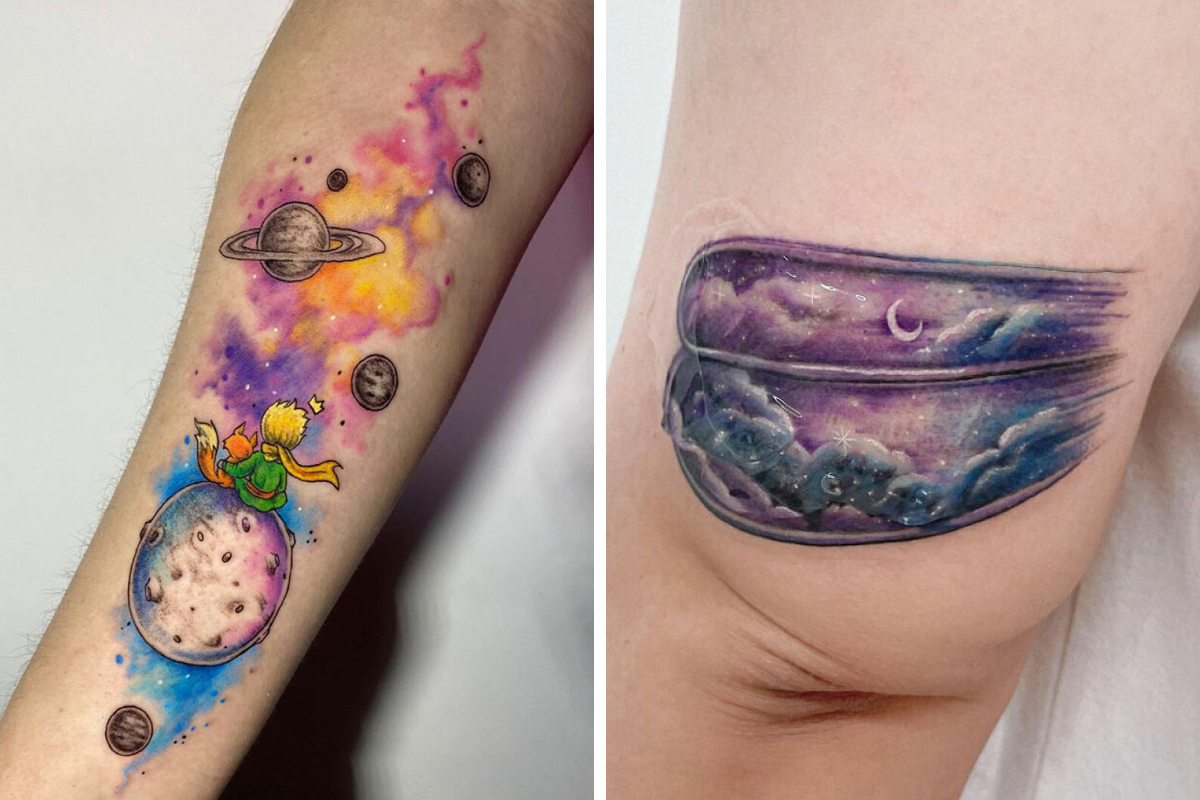The photograph features a side-by-side collage of two tattoos on the same white-skinned person. The left side reveals a detailed and vibrant inner forearm tattoo set in a colorful space scene. The background displays hues of pink, yellow, blue, and purple, with scattered white dots representing stars. Dominating this cosmic canvas is a picture of a monochrome gray planet with craters, where a young character and an orange fox sit, backs turned to the viewer. The child, adorned in a green outfit and a billowing yellow scarf, has a tuft of blonde hair resembling a wheat strand, while a whimsical yellow crown floats above their head. The child, with a left arm gently embracing the fox, gazes at the cosmic wonders. Surrounding them are additional gray celestial bodies, including a button-sized planet below them, another planet to the upper right, and Saturn with its iconic rings situated to the upper left. The overall scene also evokes the swirling pattern of smoke rising from a genie bottle.

On the right side, the tattoo depicts a serene night sky on either the back of an arm or possibly a knee. The main focal points are a large crescent moon and surrounding puffy clouds rendered in shades of purple and dark gray. The scene is framed by what appears to be two metallic, chrome-like borders that mimic the curved wrap of a car fender, with the lower border being slightly thicker. 

Both tattoos emphasize rich, vibrant colors and intricate details, capturing the viewer's imagination with their imaginative and ethereal depictions.